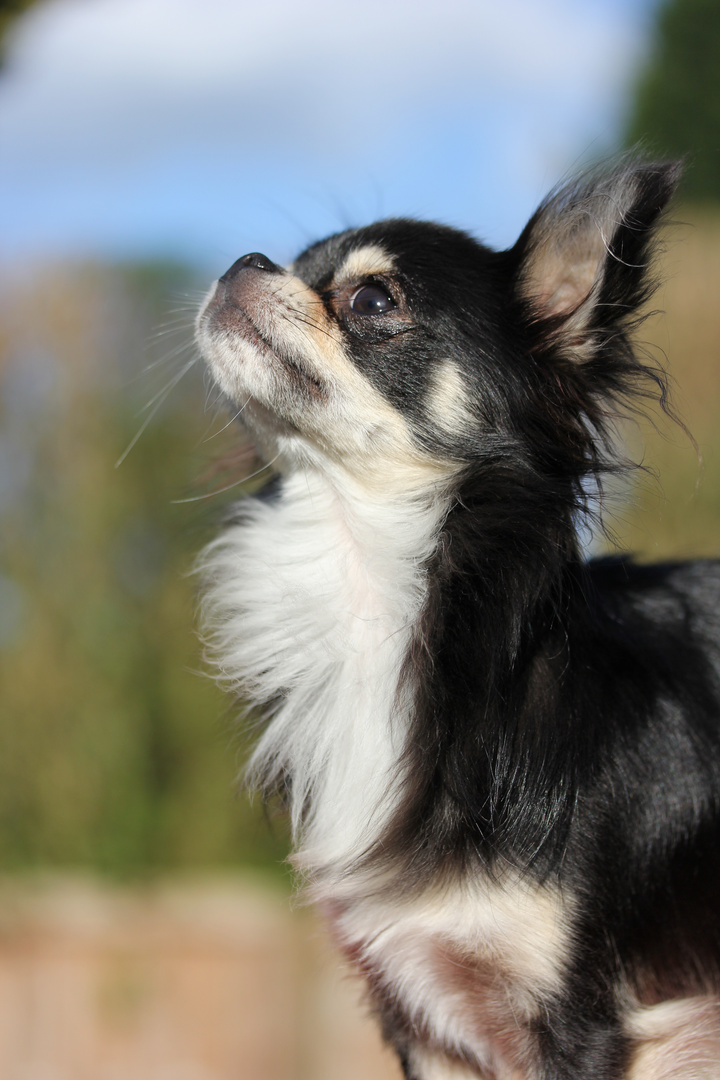The image captures a close-up view of a long-haired Chihuahua with predominantly black fur on its back and torso. The dog's face is a mix of black, white, and some brown and yellow hues, with detailed white fur around its cheeks, chin, and chest, extending to its shoulder blades. The Chihuahua has a short snout, beady dark brown eyes, and noticeable white whiskers. Its large ears appear proportionally bigger compared to its head. The dog is looking upwards, seemingly towards something out of view. The background, although blurry, reveals a clear blue sky with some clouds and green trees, suggesting that the photo was taken outside on a clear day. The lower part of the image hints at some brown ground or foliage.